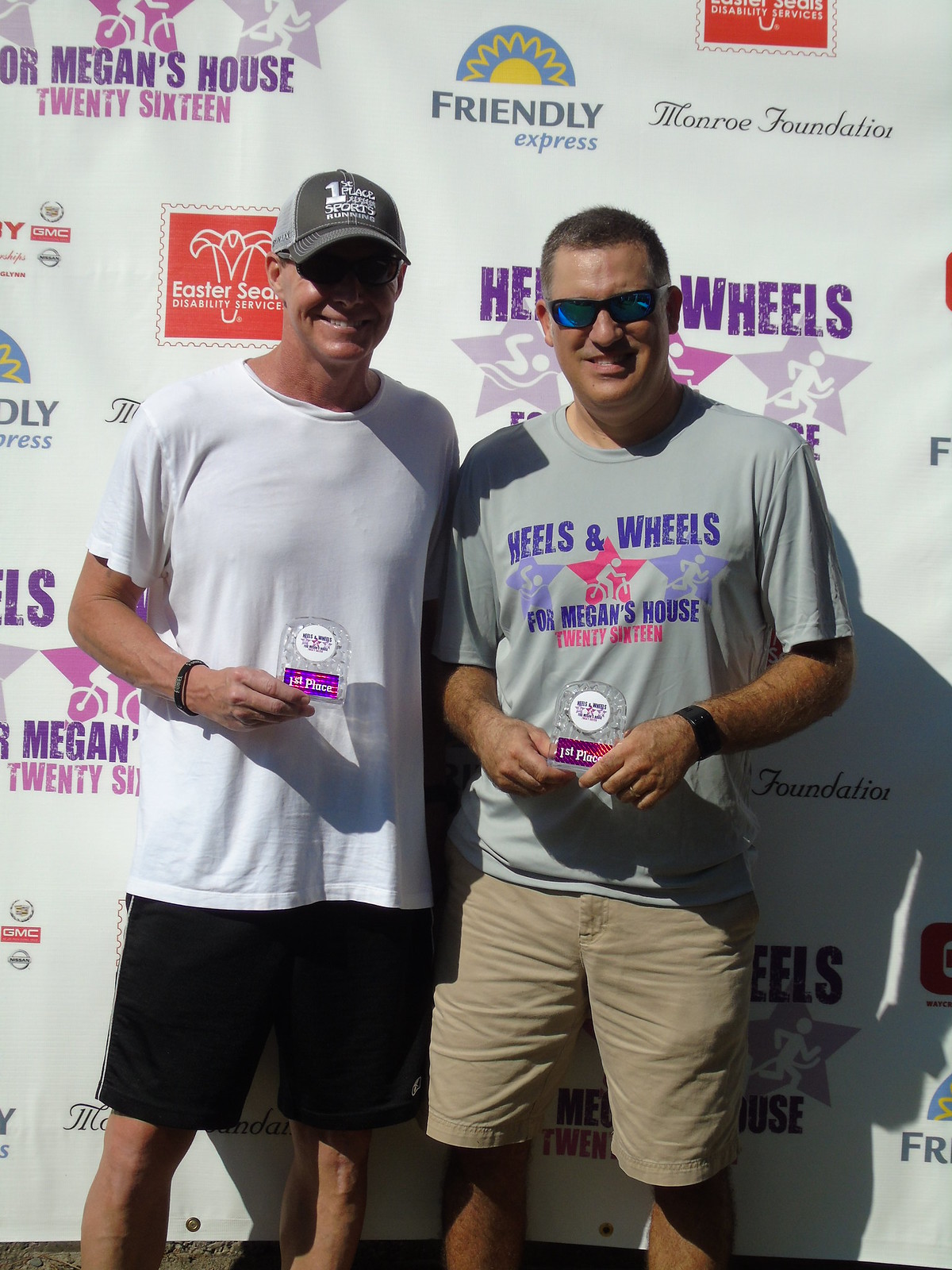Two men are posing together in front of a white backdrop covered with various sponsorship logos like Friendly Express, Monroe Foundation, Megan's House 2016, Easter Seals Disability Services, and GMC, though some logos are partially obscured. The man on the left is wearing a white t-shirt, a gray cap that reads "First Place Sports Running," and black shorts. He has sunglasses with a blue tint and something on his wrist. The man on the right has brown hair, and he is wearing a gray t-shirt featuring a graphic that reads "Heels and Wheels for Megan's House 2016," with illustrations of a swimmer, a cyclist, and a runner on three stars. He is also wearing khaki shorts. Both men are holding small trophies with first place inscriptions shaped like a circle on top of a base. The sun is shining brightly, adding a cheerful atmosphere to the photo.